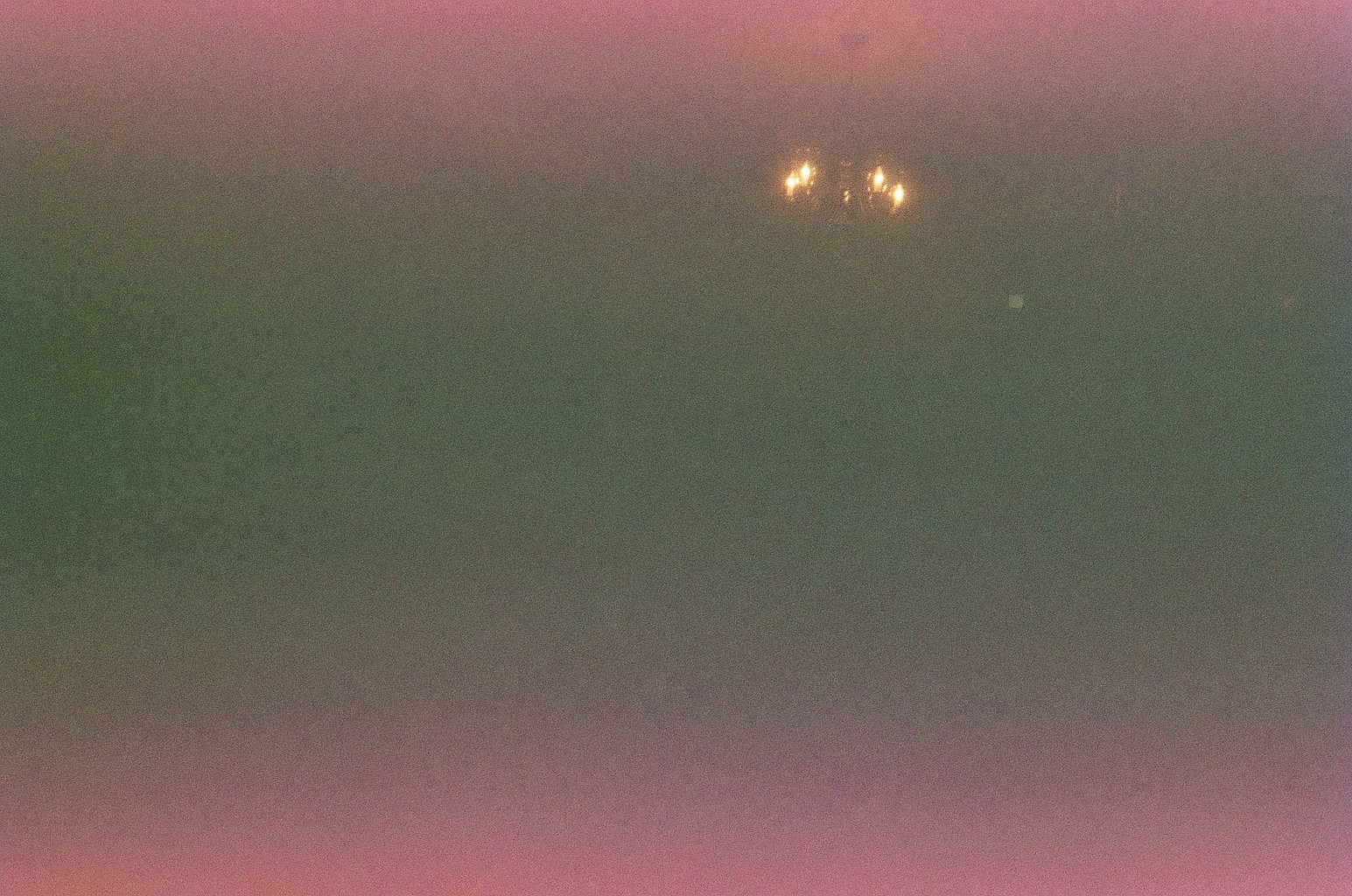A hazy, low-resolution photograph captures a mysterious nighttime scene, enveloped in dark gray and greenish tones. The image is accentuated by pink gradients at the top and bottom, adding an eerie glow. Towards the upper right corner, partially immersed in the pink hue, a chandelier with four barely discernible lights is the sole visible object, casting a faint illumination that struggles to pierce through the dim surroundings. The indistinct details contribute to an enigmatic and haunting atmosphere.